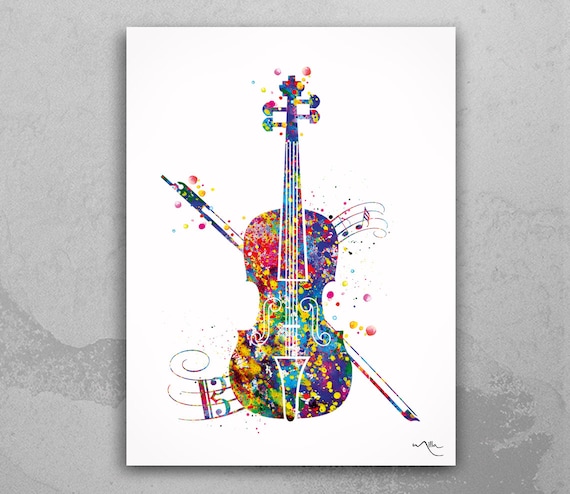This photograph captures a painting prominently displayed at the center, set against a light grey, gritty-looking background that resembles the wall of an art gallery. The painting, rendered on a white canvas, showcases a vividly colorful and large string instrument—most likely a violin—alongside a disproportionately large bow. The violin is detailed with vibrant, highly saturated hues including blues, golds, purples, reds, and pinks, evoking a lively disco effect. Adding to its intricacy, sheet music unfurls from the bottom left and top right corners of the violin, adorned with yellow, blue, green, purple, and pink paint splatter that covers the entire canvas, including the instrument and bow. The splattered colors and droplets spread across the artwork create a dynamic and uplifting visual, making it a piece that could effortlessly adorn the home of a musician.